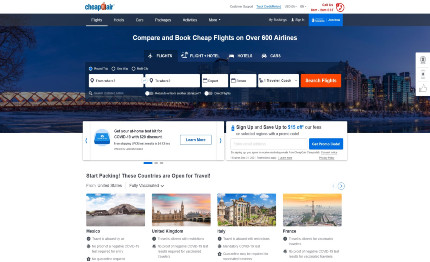The website appears to be a platform for booking affordable flights, possibly named "Cheap Air." At the top of the homepage, there's a prominent banner featuring a captivating night-time cityscape. This image showcases a long, illuminated structure, resembling a walking bridge or tunnel, stretching across a body of water.

Centrally placed within this photograph are five search bars designed for users to input their travel destinations and dates. Adjacent to these search bars, an eye-catching orange button invites users to browse available flights. A statement nearby promotes the platform’s extensive range, boasting that users can compare and book cheap flights from over 620 airlines.

Below this main section, two boxed sections draw the visitor’s attention. Each box contains a compelling statement and a button marked "Learn More." The right-hand box offers users a chance to sign up and save 15%, featuring a search bar and a blue button for easy access.

Further down the page, there is a strip of information titled "Start Packing: These Countries Are Open for Travel." This section highlights four distinct photographs from different countries, accompanied by a list explaining various travel features for each destination. The layout is designed to entice travelers to explore new locations and take advantage of the site's flight deals.